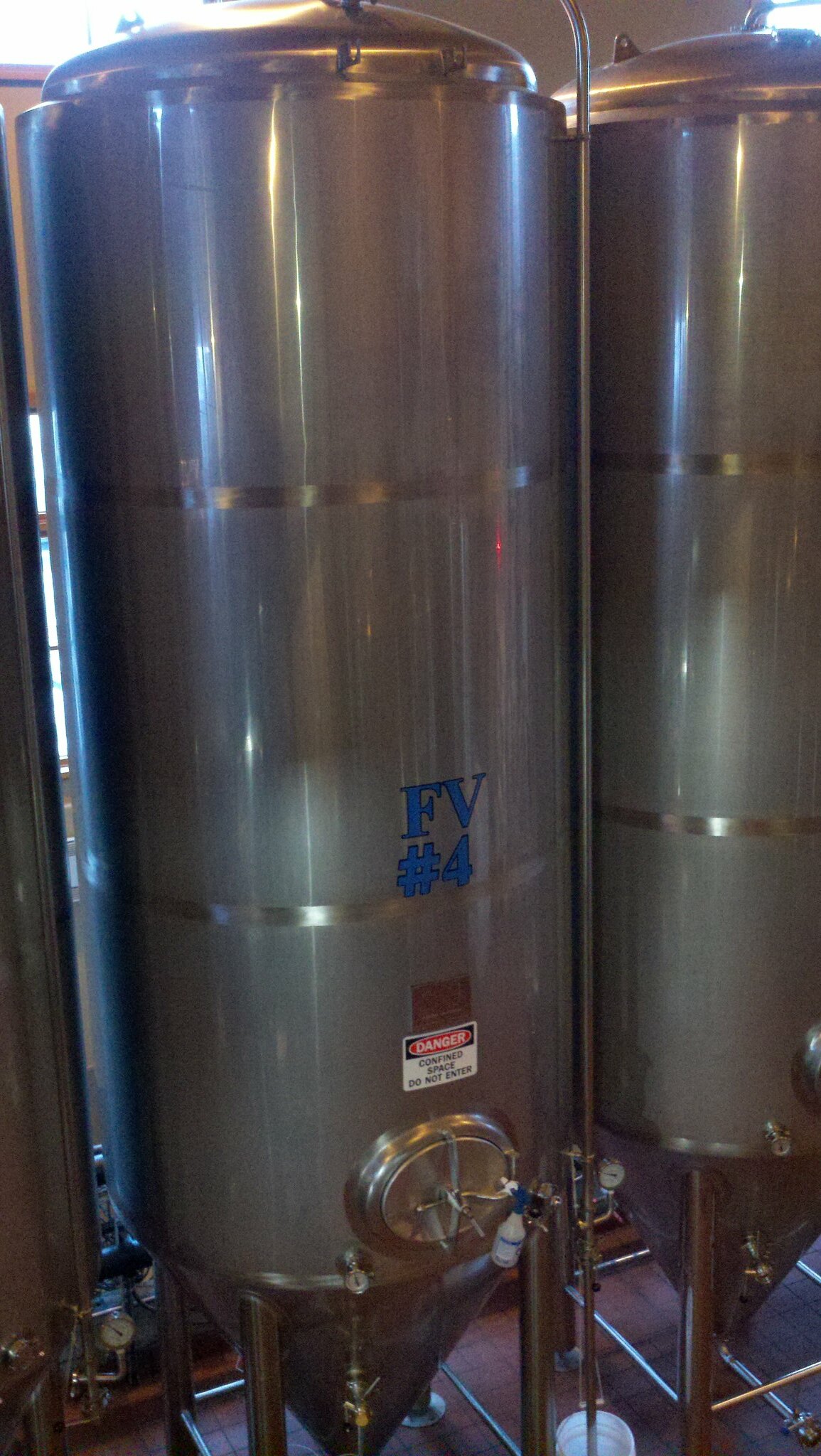The image depicts a section of what appears to be a factory or industrial setting, showcasing two large, silver containers positioned side by side. These containers resemble water heaters or distillery tanks and are cylindrical with dome-like lids at the top. Emblazoned on each tank in large blue lettering is "FV4." Directly below this identifier is a prominent warning sign with a white background and bright red text stating, "Danger! Confined space. Do not enter." Below the warning sign, there is a knob attached to a circular disc. The containers stand on slender legs and rest on a dark reddish-brown floor. The image is zoomed in, providing a detailed view of one tank while partially cutting off the one on the right. Gray pipes connect to the base of each tank, and ambient light illuminates the scene from the top left corner.